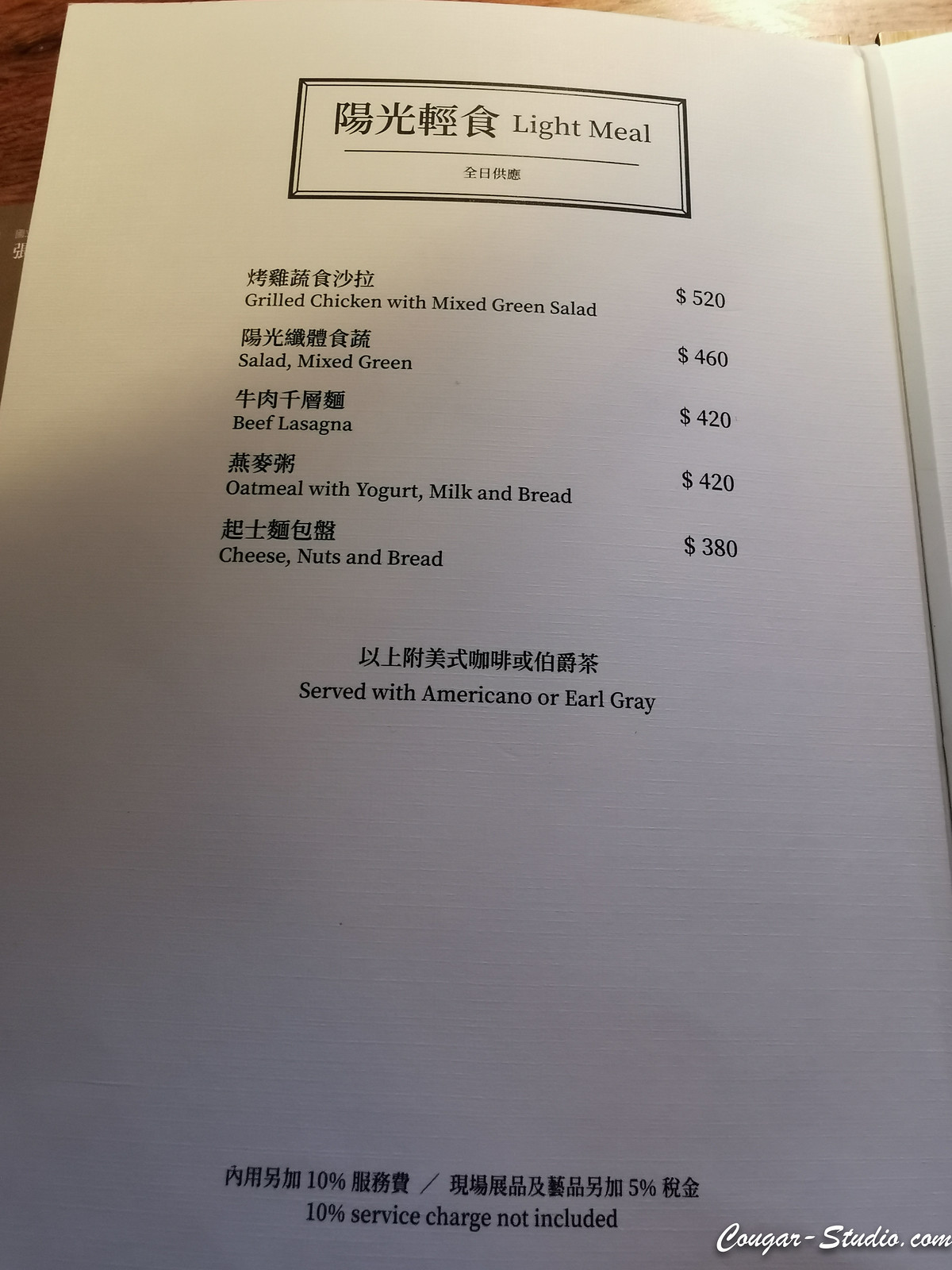This photograph captures a bilingual menu, meticulously presented in both English and an unidentified Asian script. The menu is printed on an all-white background, with a prominent black box at the top. Inside the box, encased by a fine line outline, are the Asian characters. Nearby, the words "Light Meal" are displayed in English.

Beneath this title, a horizontal line separates the heading from the actual menu items. Each menu item is accompanied by its corresponding price, indicated with a dollar sign. Here are the detailed menu listings:

1. Grilled Chicken with Mixed Green Salad ($520)
2. Salad, Mixed Green ($460)
3. Beef Lasagna ($420)
4. Oatmeal with Yogurt, Milk, and Bread ($420)
5. Cheese, Nuts, and Bread ($380)

The menu mentions that each item is served with a choice of Americano or Earl Grey tea, and it notes that a 10% service charge is not included in the listed prices.

Above each English description and price, the corresponding Asian script is displayed, maintaining a consistent bilingual format throughout the document. The bottom-right corner of the menu includes the text "Cougar-Studios.com" in white, marking the creator or designer of the menu.

This menu combines minimalist design elements with clear, bilingual descriptions, catering to a diverse clientele.